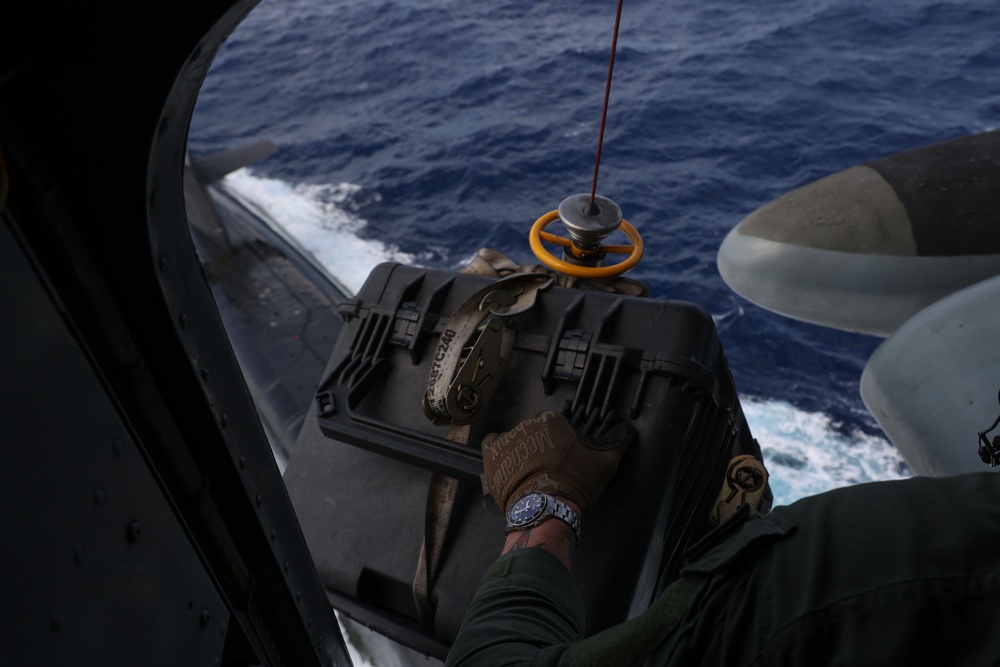This horizontal, rectangular photograph captures a close-up scene likely taken from a boat or an aircraft, such as a helicopter or carrier. In the bottom center of the image, a man's left arm, clad in a long-sleeved black shirt and wearing a brown glove, is prominently visible. He's holding onto a black handle attached to a metal wire, possibly part of a winch or crane system, suggesting that the object was recently lifted from the water. The object he's gripping resembles a locked army chest or cooler. The scenery behind him features the wavy blue expanse of the ocean, and on the right side, an orange-colored wheel with a red pole protruding from it is partially visible. Additionally, there's a small glimpse of what appears to be a shoe sticking out of the frame on the right. On the left-hand side, there’s a curved edge resembling a window or door frame, indicating the photo might have been taken from an opening. The scene is immersed in the deep navy blue of the water, further highlighting the marine or aerial nature of the environment.